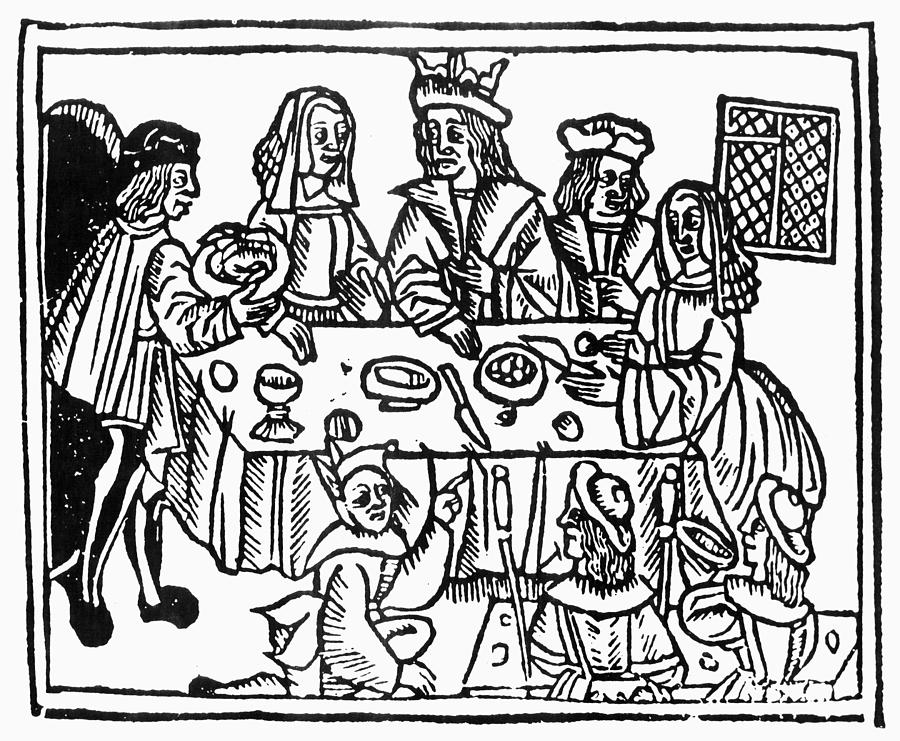The image is a detailed black-and-white drawing depicting a medieval family scene at a dinner table. The central figure, a king, is identifiable by his regal robe and crown, and is surrounded by his court. The king sits at the center of the table, covered with a white cloth, which holds numerous bowls, cups, pieces of silverware, and various fruits. To the left of the king is a woman, possibly the queen, adorned in a long-veiled headdress. On the right side, a man with a concerned expression points to the right, while another person appears to be waiting or in deep thought. In the foreground, a jester and two other people sit on the floor by the table. On the table itself, there are three bowls and two knives. 

A man wearing a long-sleeved outfit with a cape is seen entering from a doorway on the far left, carrying a platter, possibly with a turkey or bird. The background features a small lattice window on the right side of the image. The entire drawing is framed with a white border and is devoid of any text.